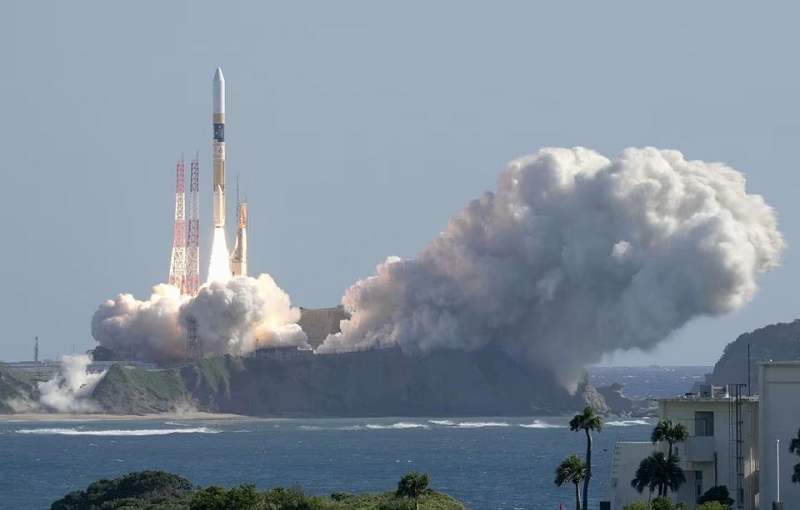The photograph captures a dramatic rocket launch taking place on a small island or peninsula, surrounded by a body of water with a rocky shoreline. The launch pad is equipped with two red and white towers that seem to have supported the slender, pencil-like rocket. The rocket, yellow and white at its base, is half-way into its ascent, trailing a vast plume of thick, white smoke that billows to the right, with occasional gray shades due to the lighting. The rocket's base emits fiery bursts of yellow and white flames, indicating intense propulsion. 

In the foreground, beyond a stretch of water, a bit of vegetation is visible, including trees and some small, squarish white buildings, possibly housing facilities or equipment, with poles, wires, and an air conditioning unit on one of the roofs. The scene captures the raw power and engineering of space exploration, all set under a gray, neutral sky.